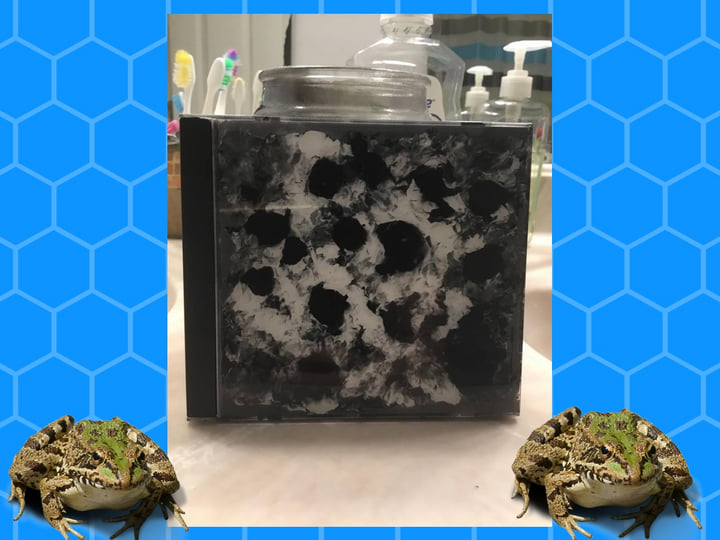This image is a wide rectangular digital artwork featuring a central photograph that captures a CD propped against what seems to be a jar candle on a bathroom counter. The setting includes a sink to the left, toothbrushes, hand soap, and a bottle of mouthwash, providing a domestic backdrop. The CD is encased in a jewel case with an abstract black and white design, resembling an oil painting with black dots on a white backdrop and a black border. Surrounding this central photograph is a frame with a blue background adorned with dark blue hexagon shapes, thicker on the left and right sides. At the bottom of the artwork, there are two identical green frogs with dark green stripes and white underbellies, each one overlapping slightly with the left and right edges of the photograph, adding an eclectic touch to the composition.